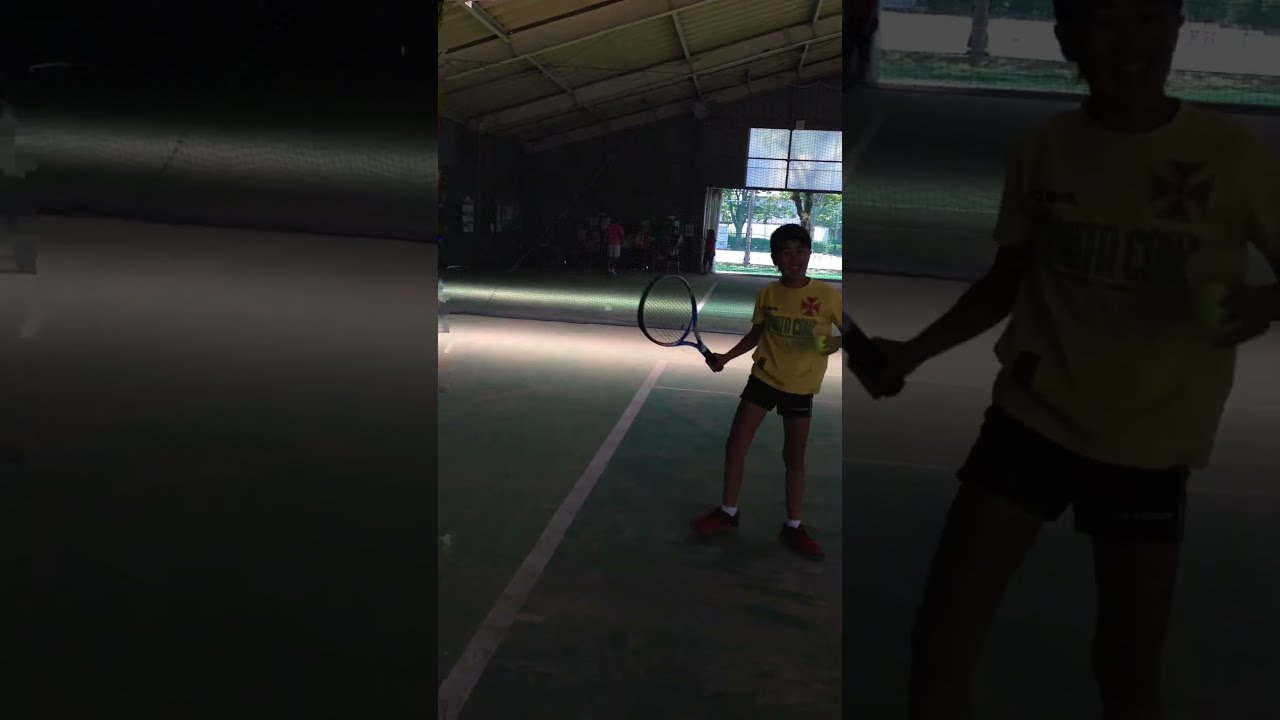The image portrays an indoor tennis court with a distinct split layout, where both the right and left sides are darkened panels. At the center of the image stands a young boy dressed in a yellow shirt featuring blue text and a red cross, complemented by dark shorts, short white socks, and black shoes. In his right hand, he holds a black and blue tennis racket, and in his left, a tennis ball. He faces outward with both arms close to his body. The indoor environment, potentially a gymnasium, has a lighter center area under some lights, and a darker perimeter. The court floor is a mix of dark and light green with white lines, and the ceiling, adorned with white or gray and silver bars, slopes at an angle. In the background, a large rectangular window reveals green trees with brown trunks, an expansive lawn, bushes, and a possible body of blue water outside. A group of people, consisting of both adults and children, is gathered in a dimly lit corner of the indoor space.